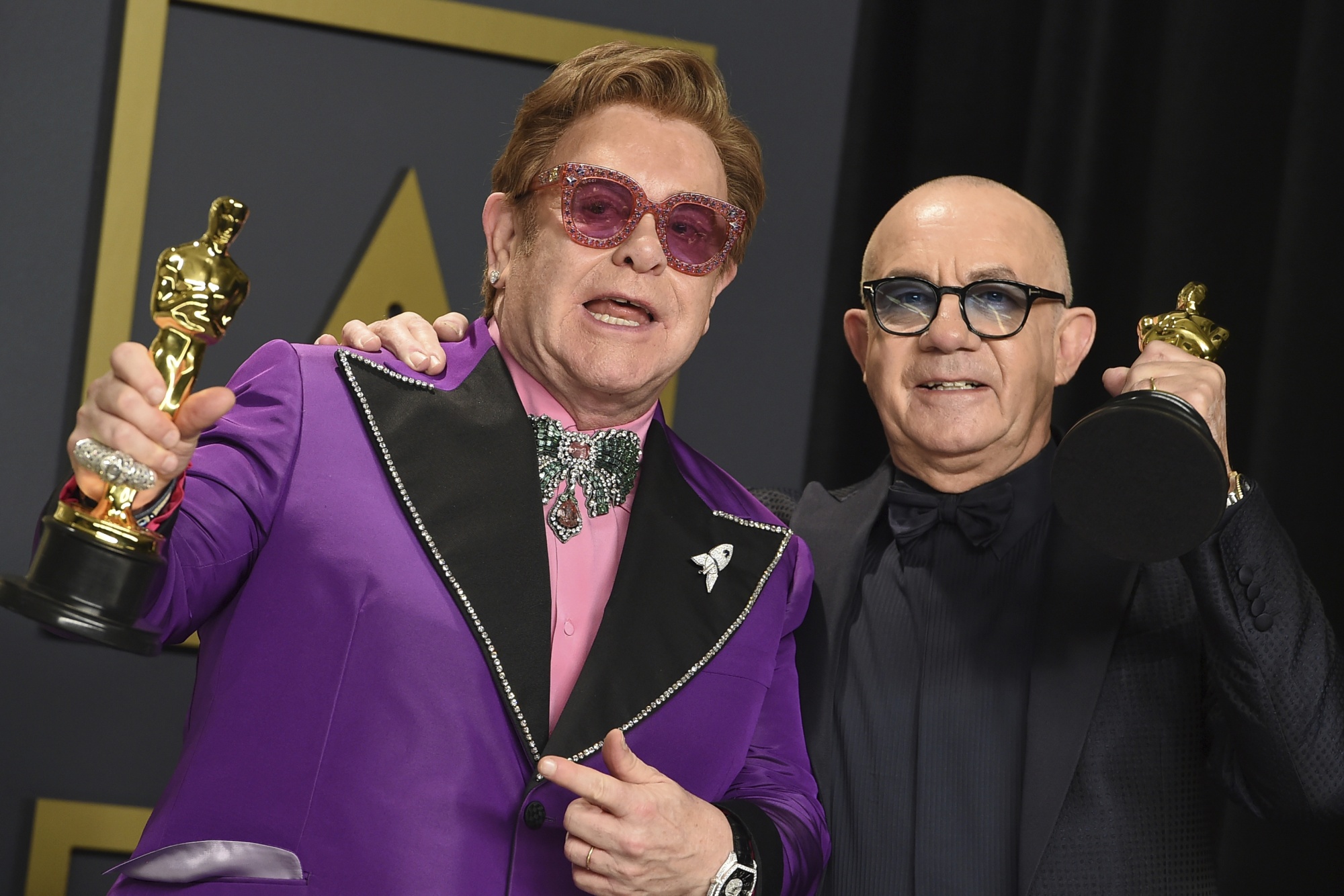The photograph depicts Elton John and Bernie Taupin at an awards ceremony, likely the Grammys or Oscars. Both men are captured from the waist up, posing for the camera with golden statuettes in their hands, each resembling a man on a black base. Standing against a backdrop featuring a gray wall with a golden square design and black curtains, the two share a visually engaging and celebratory moment.

Elton John, on the left, sports a vibrant purple suit jacket adorned with wide black lapels decorated with silver beading. Underneath, he wears a pink collared shirt with intricate appliques and jewels. His large, jeweled-framed glasses with pink-tinted lenses add a flamboyant touch to his look. Elton's dyed brown hair is short and curled, and he gestures animatedly with his left hand while holding his award in his right.

Beside him, Bernie Taupin exudes a more subdued elegance in an all-black tuxedo with a black bow tie. He is bald, wearing black-rimmed glasses with a bluish tint at the top. Bernie holds his trophy over his shoulder, mirroring Elton's pride. Behind them, the contrasting backdrop of black curtains and the gray wall with its distinctive golden design frame the scene perfectly, highlighting the significance of their achievement.